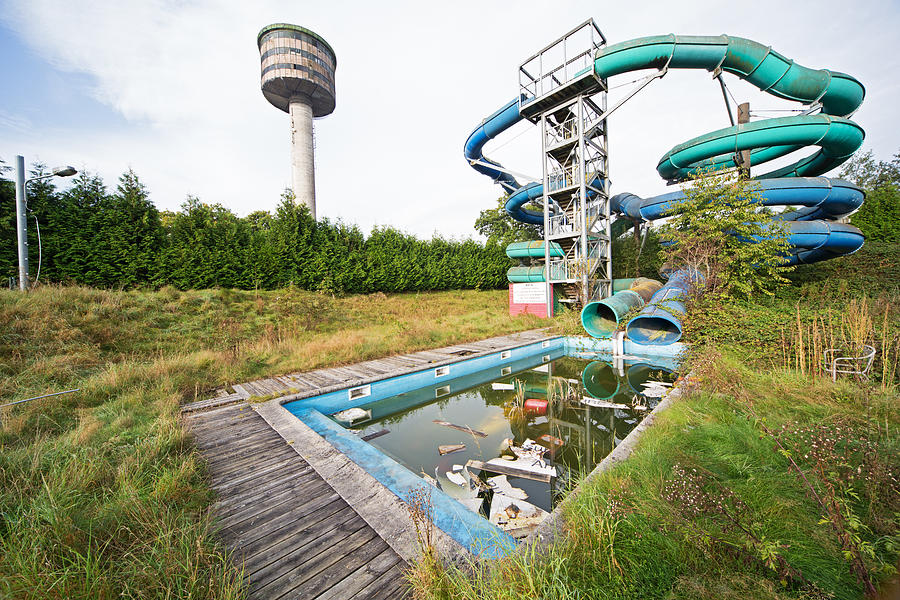This photograph showcases an abandoned water park set against a sky partially covered by large, white, puffy clouds with glimpses of blue breaking through. The scene is dominated by a murky, greenish-brown pool filled with floating debris and garbage, hinting at its disuse. Spanning the pool, a green and blue water slide spirals, each section veering in opposite directions before emptying into the filthy water. The slide, with its worn appearance, is accessed via a white tower with stairs. Across the landscape, patches of both green and brown grass are visible, along with a weedy, white-framed chair on the far right. Surrounding the area, dark green hedges and shrubs form a border, giving way to a distant, crow's nest-like structure made of wood with a white base. Adding to the eerie abandonment, a tall tower with a circular top and brown windows stands tall to the left, against a backdrop that merges nature’s overgrowth with dilapidated, man-made fun.